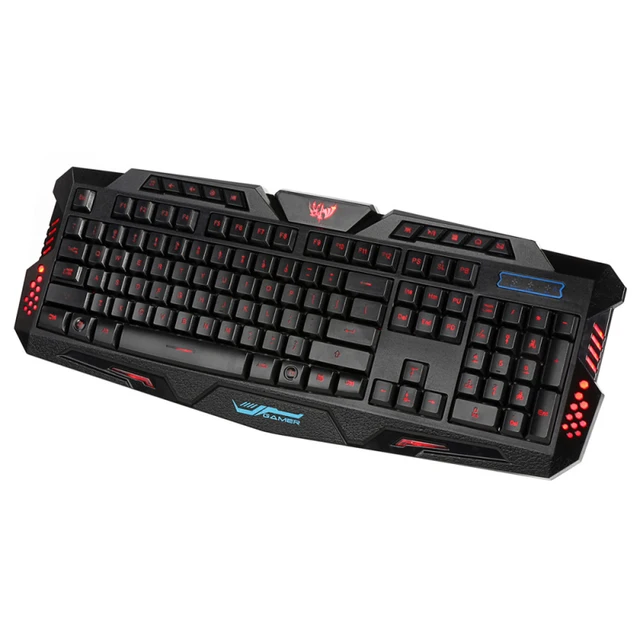Centered against a solid white background, this image prominently features a large, modern computer keyboard designed for gamers. The rectangular keyboard is primarily black and boasts a sleek, futuristic appearance. It is adorned with a variety of colors, including black, red, light blue, and dark blue. The keys are black with red icons and symbols, and the word "gamer" appears in light blue with accompanying symbols above and beside it. 

Red LEDs illuminate parts of the keyboard, with glowing dots on the right, near the number pad, and on the left, below the shift key. A red flame design decorates the top center area of the keyboard. Additional design features include a standard QWERTY layout, a number pad on the right, function keys situated to the left of the number pad, and extra keys above the function keys for various tasks.

The absence of any extra text apart from the keys' letters suggests that this image could be used in a product advertisement or as a showcase of someone's owned keyboard. The keyboard appears to be in excellent condition and well-positioned, taking up almost the entire image and directly centered within the frame.